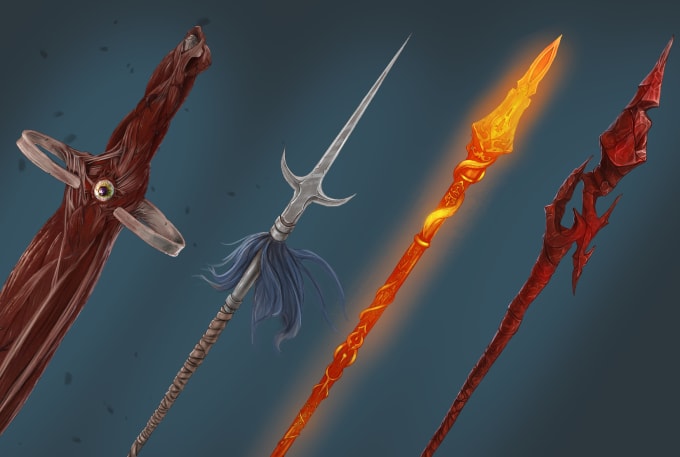The image portrays a detailed artwork featuring four diverse weapons set against a dark, cobalt blue background adorned with black spots. The weapons, arranged diagonally from the lower left to the upper right, each exhibit unique characteristics. The weapon on the far left resembles a spear crafted from a blend of muscle and skin-like textures, culminating in an eyeball at the handle junction, with bone fragments integrated into its design. Next, there is a traditional-looking spear with a metallic body accented by blue feathers at mid-length, ending in a trident-like tip with a prominent central prong. The third weapon in the sequence glows with an orange hue, showcasing ornate wrapping and a flat yet pointed end, evoking the image of meticulously forged metal. The final weapon on the right appears to be a staff or spear made from red crystalline material, characterized by its jagged, sharp edges and a tapering pointed tip. The overall two-dimensional, almost cartoonish illustration style further enhances the distinct and imaginative nature of each weapon.